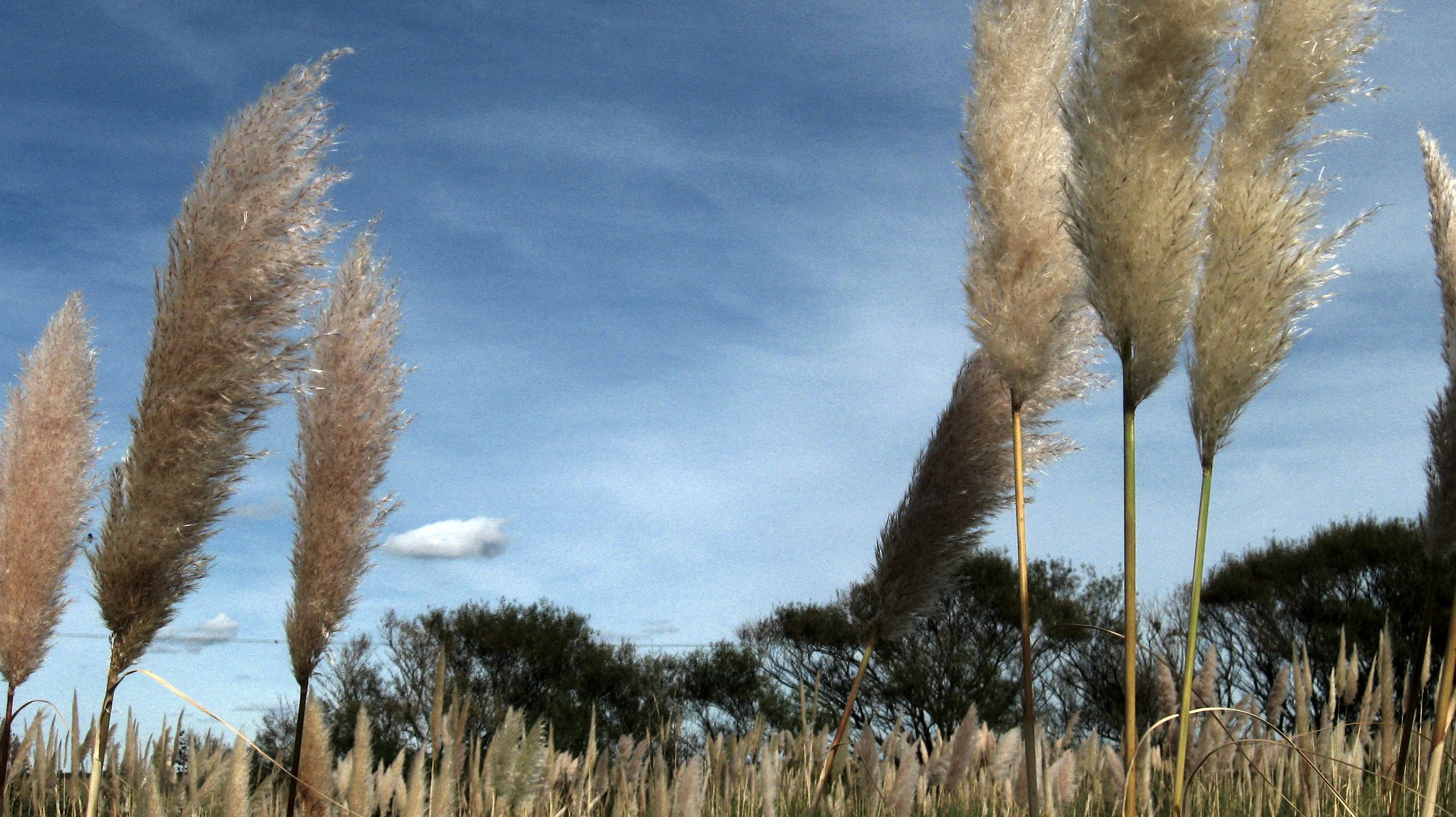In this detailed outdoor nature photo, captured from ground level, we see a dense field of pampas grass stretching into the distance, with tall, silvery, and white plumes crowning golden brown stems. Dominating the foreground, several reeds stand tall and fuzzy, particularly on the right side, where five notable cattails with bushy tops appear, with three being closest to the camera and the tallest. On the left side, three more reeds rise, with the nearest one being especially long. Beneath this foreground layer, the bottom eighth of the image is filled with more distant, shorter reeds, indicating depth. Extending across the horizon, a distant tree line spans the width of the image, dotted with dark green foliage. Above this, the upper three-fourths of the image showcase a partly cloudy sky, where light blue hues intermingle with thick, fluffy white clouds, particularly congregated on the left side. Overall, the photograph, taken at the height of the reeds, emphasizes the lushness and expansive nature of the pampas grass field against the serene, cloudy sky.